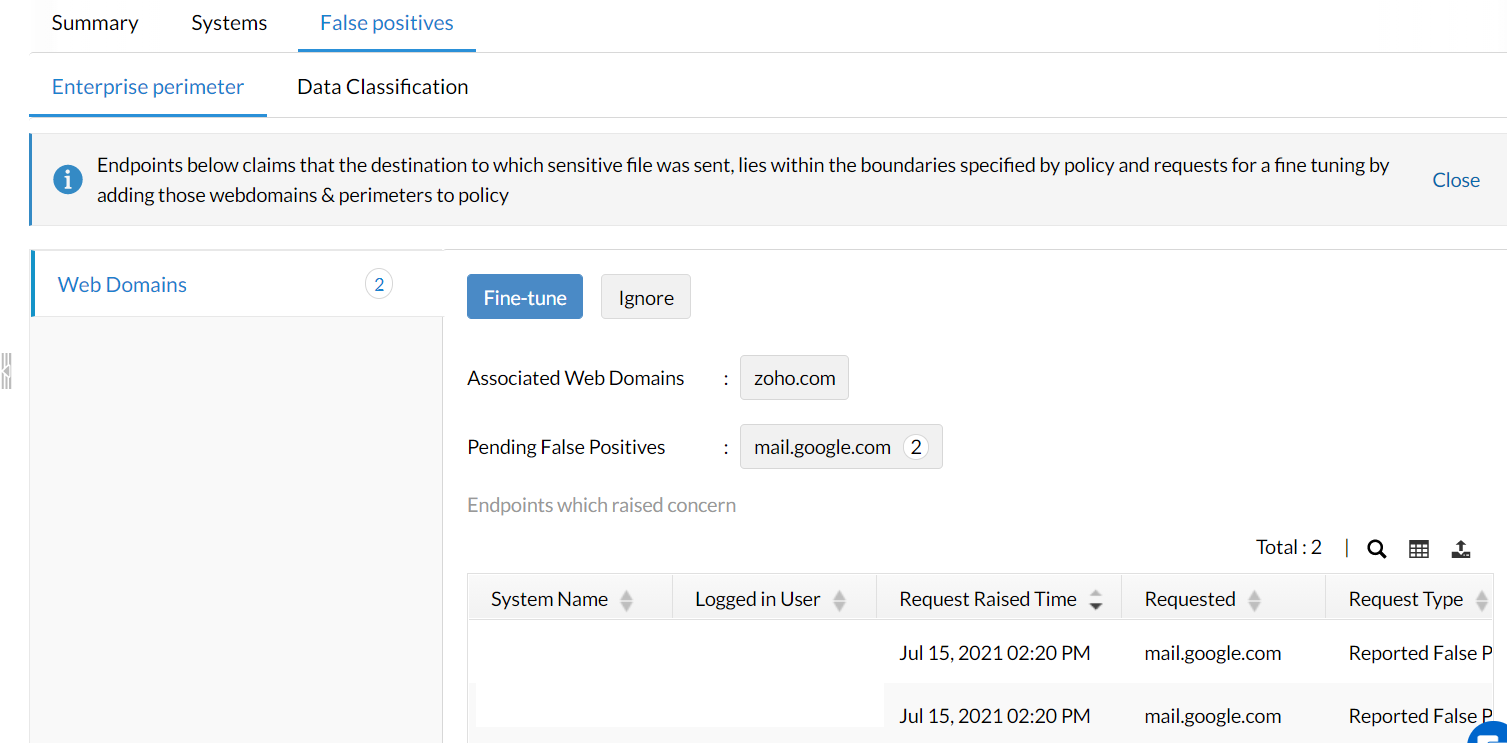A sophisticated control dashboard is depicted in the image, showcasing various analytics and system summaries. The dashboard, set against a gray background, features sections labeled "Summary Systems," "False Positive," "Expertise Perimeter," and "Data Classification." It meticulously lists numerous web domains accompanied by detailed information such as the logged-in user, system name, type of request, and timestamps, indicating a timeline of activities. Prominently displayed are actionable buttons, including a blue "Fine Tune" icon and a gray "Ignore" icon, suggesting user interaction capabilities for domain management. This comprehensive dashboard provides a robust overview of domain-related activities and system statuses.